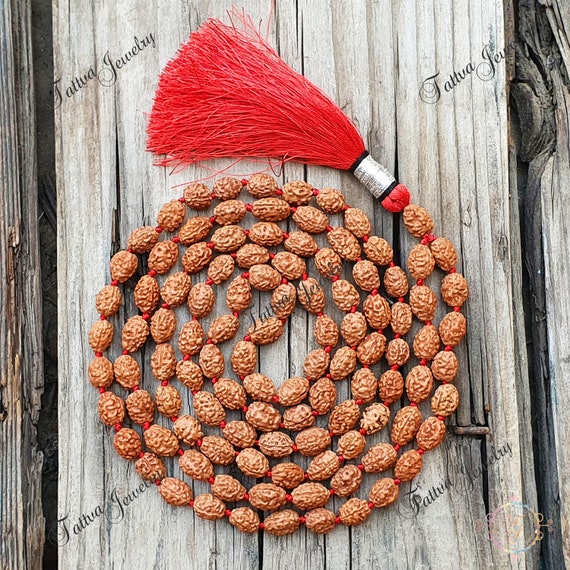This image showcases an intricate piece of jewelry, prominently featuring a string of knotted, textured brown beads resembling walnuts, artfully arranged in a spiral formation on a rustic, handmade wooden surface. The beads are interspersed with small knots along a vibrant red string and culminate in a striking red tassel accentuated with silver thread. The backdrop of rough planks adds a natural, handcrafted charm to the composition. Overlaid across the image multiple times is the scripted watermark "Tatva Jewelry," suggesting the brand's presence, with a partially visible, multi-colored emblem in a pastel circle adorning the bottom right corner. The writing intertwines with the photographic elements, crafting an elaborate and detailed portrayal of this unique jewelry piece.